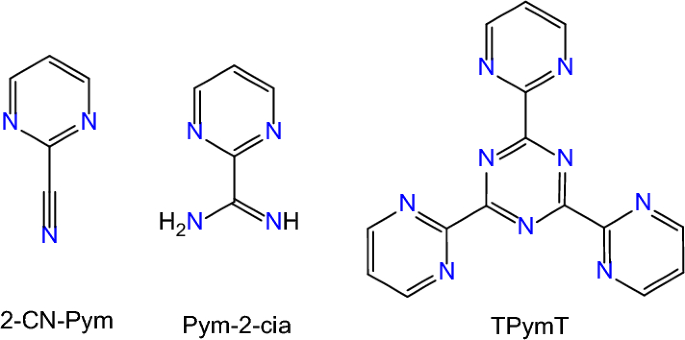The image displays a detailed schematic of three chemical compounds, each represented by distinctly structured elements. On the left, the compound labeled "2-CN-PYM" features a pentagon-shaped top with blue corners. Below the pentagon, a straight line descends, splitting into three small vertical lines. The central compound, labeled "PYM/2/CIA," continues with the same pentagon and blue corners design, however, the descending line forks into two sections, labeled "H2N" and "NH" in black. The final compound on the right, labeled "T-PYM-T," features a more complex structure with a central element and branches consisting of one element on top, one in the middle, and two on each side. All nitrogen elements within these compounds are depicted with blue characters, and the background is white.